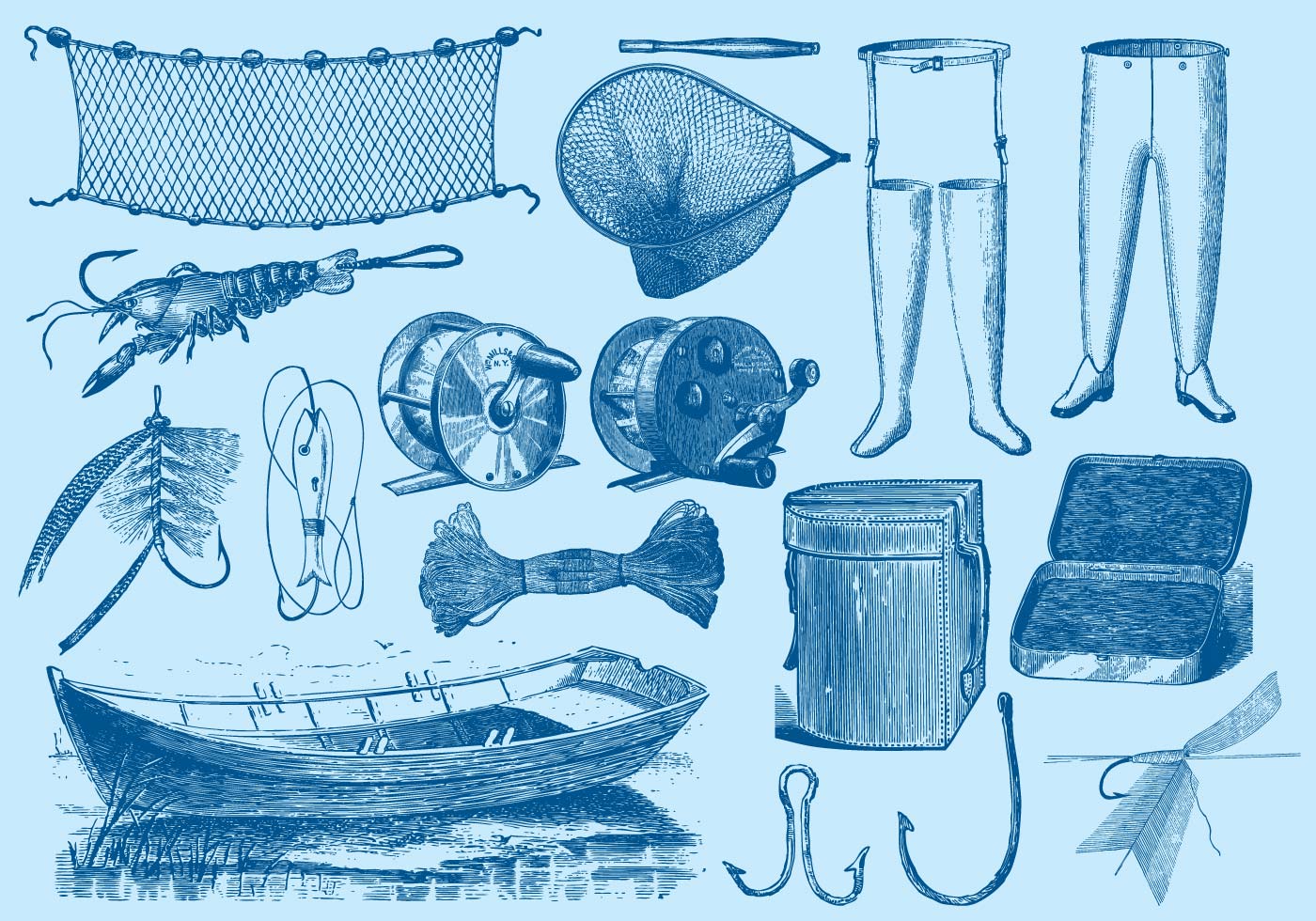This image is a detailed illustration showcasing various fishing equipment, depicted in dark blue sketches on a light blue background. The top left features a fishing net, and directly beneath it is a lobster. Adjacent to these are two types of fishing lures and a couple of reels, essential for fishing lines. At the center, a hand crank for fishing poles is prominently displayed. 

A small, rowboat with fronds poking out of the water rests in the bottom left corner, designed with two fishing mounts on each side. Nearby, there's a bundle of twine and a bait bucket. Towards the right, two pairs of rubber waders designed to keep fishermen dry are visible, next to a net basket. Further down, a little tin with its lid open, possibly for lures, can be seen. 

The bottom right corner includes a variety of hooks, including a double-sided hook and a fly fishing lure. Together, these objects form a comprehensive and cohesive collection of fishing gear, all intricately sketched to highlight the essentials of a fishing operation.